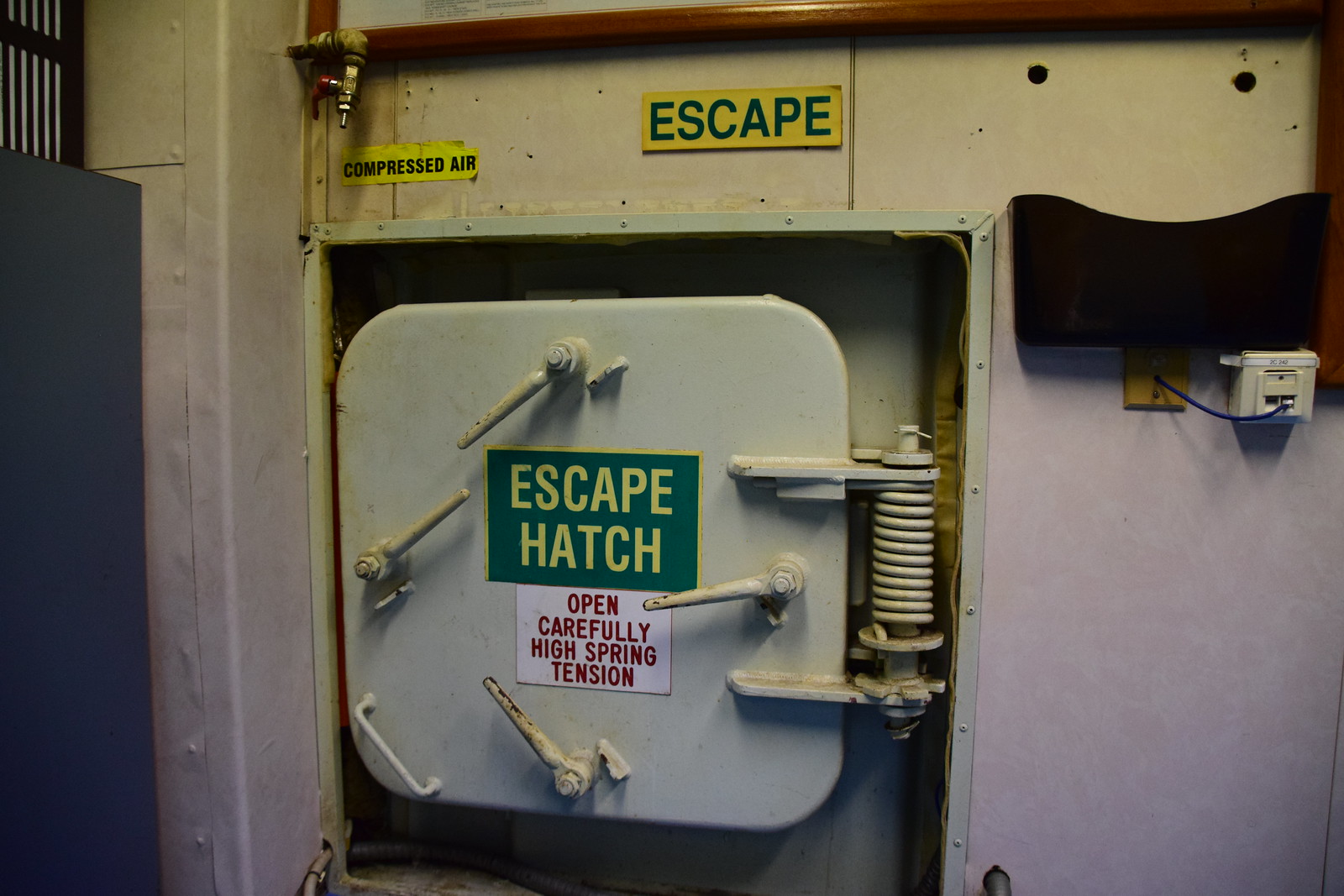In this detailed close-up image taken inside an industrial facility or factory, the focal point is a metal escape hatch prominently labeled with a green rectangular sign that reads "ESCAPE HATCH" in yellow letters. Below this sign, there is a white sign with red lettering that warns, "OPEN CAREFULLY, HIGH SPRING TENSION." The hatch itself features multiple valves and handle levers, essential for its operation. To the right of the hatch, a large, robust spring is visible, emphasized by its installation which supports the high tension mechanism.

Directly above the escape hatch, there is an inverted yellow rectangular sign with green lettering that reads "ESCAPE." Slightly to the left, another yellow background sign, this time with black capital letters, indicates "COMPRESSED AIR," and a nozzle can be seen above this sign. To the right of the hatch, a blue wire runs out from an outlet on a white wall, and there's a black container-like structure that looks like a jack or phone jack, affixed to the wall. The overall scene captures the complexity and functionality of industrial safety mechanisms.